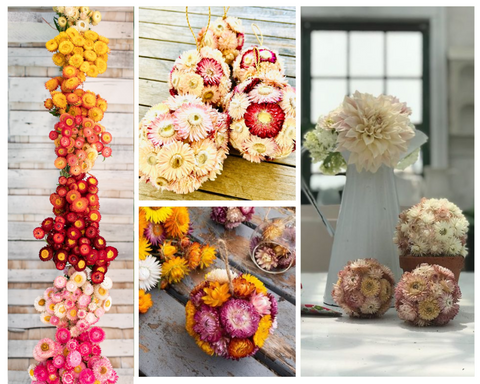The image is a square collage composed of four distinct photographs, each separated by a thin white line. On the left side, a vertical rectangular photograph showcases a vibrant column of floral arrangements, featuring round bundles of yellow, pink, dark red, light white, and hot pink flowers, arranged in succession from top to bottom. In the top-center portion, another rectangular photograph displays five ornament-like balls made of various combinations of yellow, pink, and red flowers, each attached to a string, adding a festive touch. Below this, in the bottom-center, a similar flower ball arrangement is presented, resting on a flat wooden surface, and includes an eclectic mix of red, yellow, and white flowers. Finally, the right-side photograph highlights a pristine, white metallic watering can on a flat white table, accompanied by three flower balls created from white and light pink blooms, adding a softer, more delicate contrast to the collage.